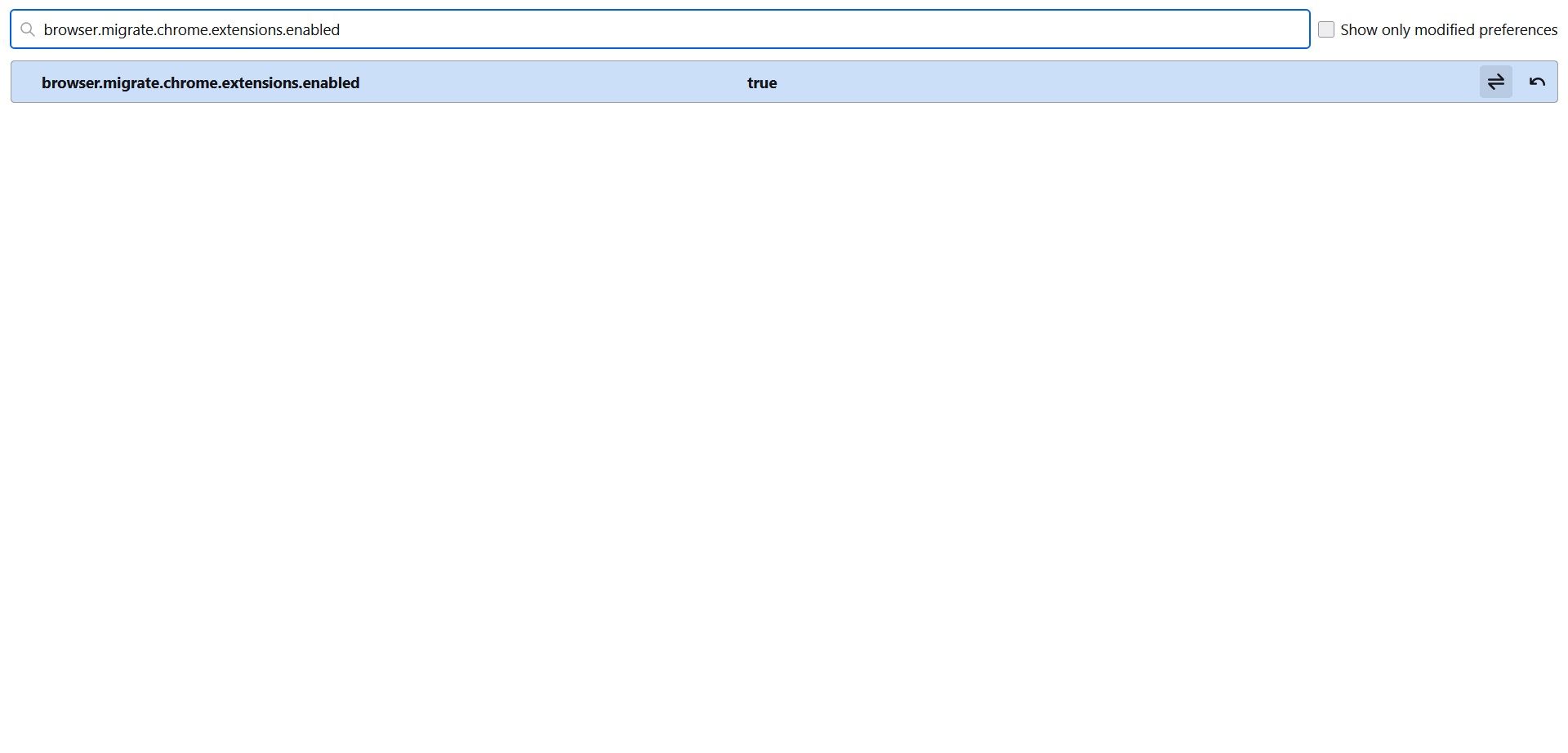The image captures a section of a Google Chrome preferences menu. The screen primarily displays the option "Migrate Chrome extensions" with an associated checkbox that is marked, indicating the feature is enabled. This text is white with a blue outline and presented alongside black lettering against a white background. Below this, there is a search bar where the text "browser Migrate Chrome extensions enabled true" appears in blue. The remaining details on the screen confirm that no other preferences have been modified. The uncluttered layout consists of concise text in black against a clean interface. There are no additional items loading, affirming that only these two specific lines are visible.